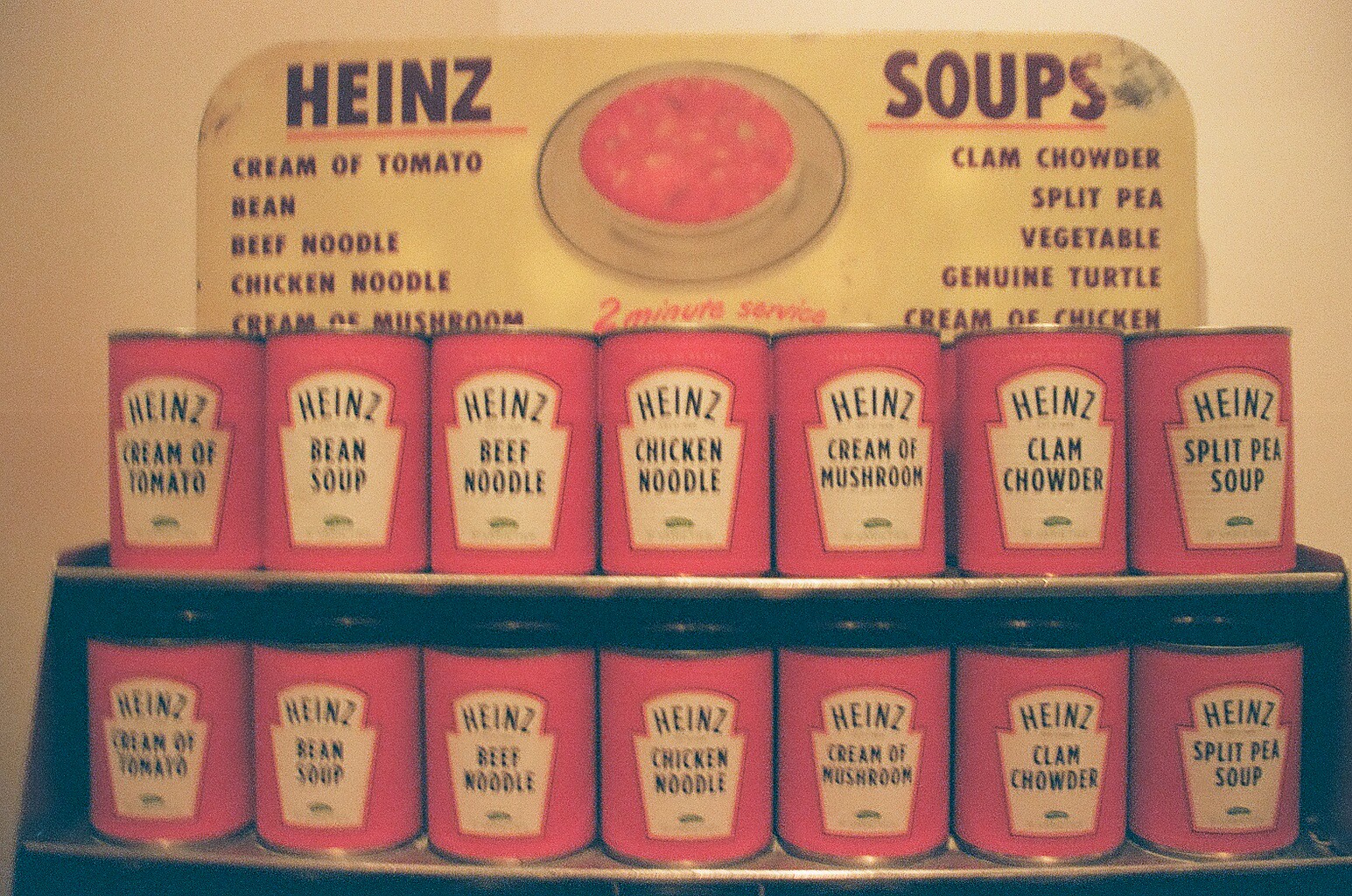This vintage photo captures an elaborate Heinz soup display. In the background, a white wall supports a black shelf filled with various Heinz canned soups. Each can, made of aluminum, is adorned with a distinct red label featuring the name "Heinz" in a white panel with black writing. The labels also indicate the type of soup, highlighting a rich assortment including Cream of Tomato, Bean Soup, Beef Noodle, Chicken Noodle, Cream of Mushroom, Clam Chowder, and Split Pea Soup. Above the shelf, a sign prominently reads "Heinz Soup," listing the different soup varieties. A central image on the sign displays a bowl of soup with the caption "Two Minute Service" underneath, emphasizing the convenience of the product.